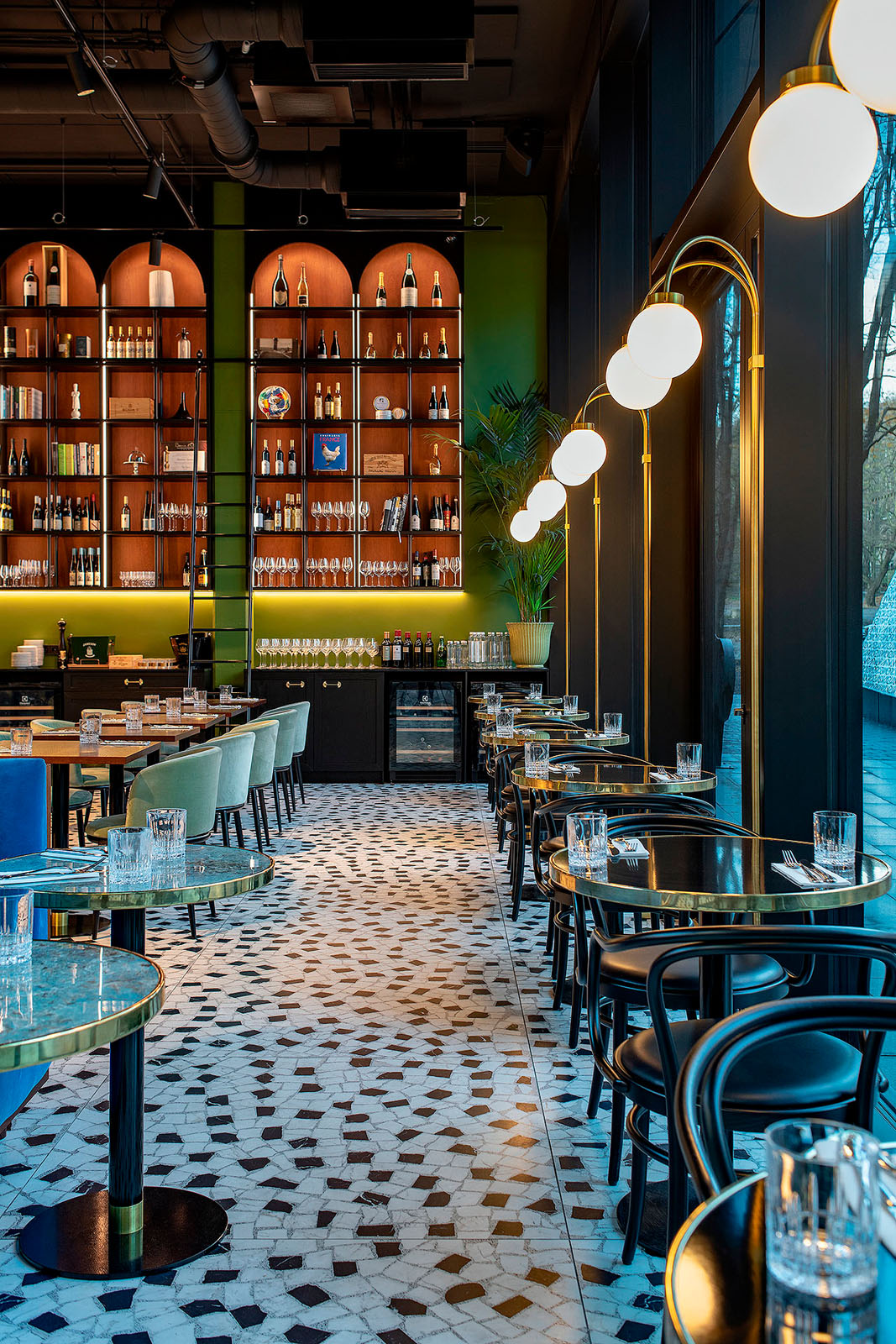The image depicts a stylish and sophisticated bar interior. Along the window side, several intimate round tables are set for two, featuring cut crystal glasses and neatly arranged silverware on folded napkins. These tables are paired with small, black, circular stools. The bar also has larger tables set for groups, outfitted with comfortable white and raised blue-backed stools. 

The bar's ambiance is enhanced by street lamp-like fixtures with round globes emitting a bright yellowish-white light, positioned between the windows and hanging from the ceiling, which is painted black but reveals the exposed industrial pipes above. The floor sports a classic black-and-white checkered tile pattern.

Dominating the back wall are very tall, arched cabinets with a rich red-orange background. These impressive cabinets have five neatly arranged shelves displaying numerous liquor bottles and glasses. At their base, the cabinets transition to sleek black shelving, with additional liquor bottles positioned on the counter. The primary wall behind the bar is painted a pleasing medium green, adding to the refined atmosphere of the space.